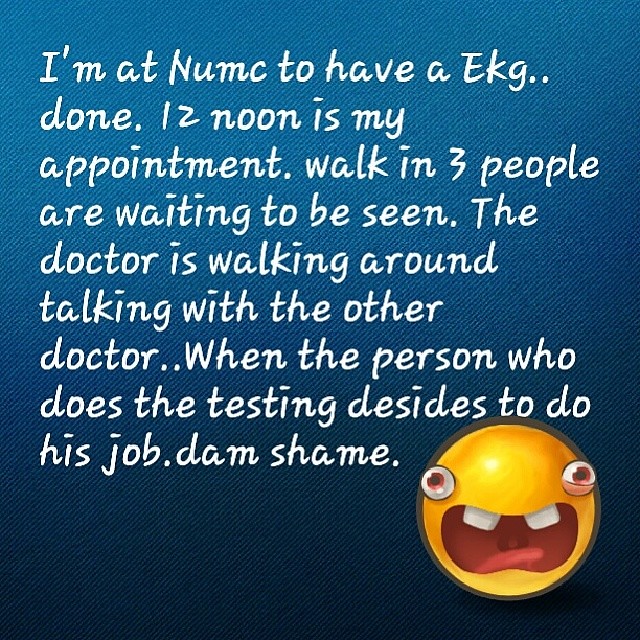The image consists of a post with white text against a gradient blue background, which transitions from a lighter shade at the top to a darker shade at the bottom. In the lower right corner, there is a cartoonish yellow emoji character. This character has bulging eyes positioned on the outer sides of its face, an open mouth showing red inside with a visible tongue and uvula, and two gapped front teeth, creating an expression that appears shocked, unhappy, or possibly screaming. The text on the image, despite containing some typos, reads: "I'm at NUMC to have an EKG done. 12 noon is my appointment. Walk in, three people are waiting to be seen. The doctor is walking around talking with the other doctor. When the person who does the testing decides to do his job, damn shame."